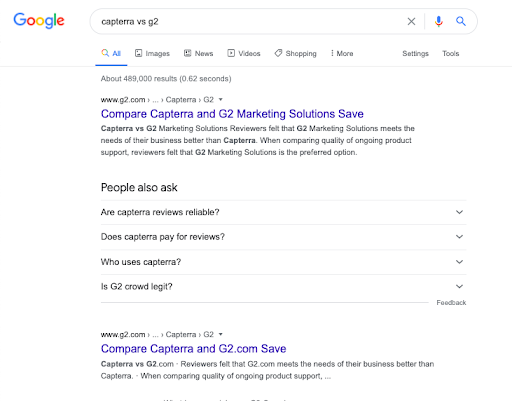The image shows a Google search results page with the query "Capterra vs G2" entered into the search bar, positioned below the iconic Google logo in the top left. Directly beneath the search bar, the standard Google search category options are visible, including "All," "Images," "News," "Videos," "Shopping," "More," "Settings," and "Tools."

The search results begin with a prominent link to G2.com, highlighting a comparative analysis of Capterra and G2 marketing solutions. The summary indicates that reviewers generally believe G2 marketing solutions better meet the needs of businesses, especially regarding the quality of ongoing product support, making G2 the preferred choice.

Further down the page, a "People also ask" section lists related queries such as "Are Capterra reviews reliable?", "Does Capterra pay for reviews?", "Who uses Capterra?" and "Is G2 Crowd legit?"

Below this, another link to G2.com appears, reiterating the comparison between Capterra and G2, once again noting that G2 is favored by reviewers for its superior product support.